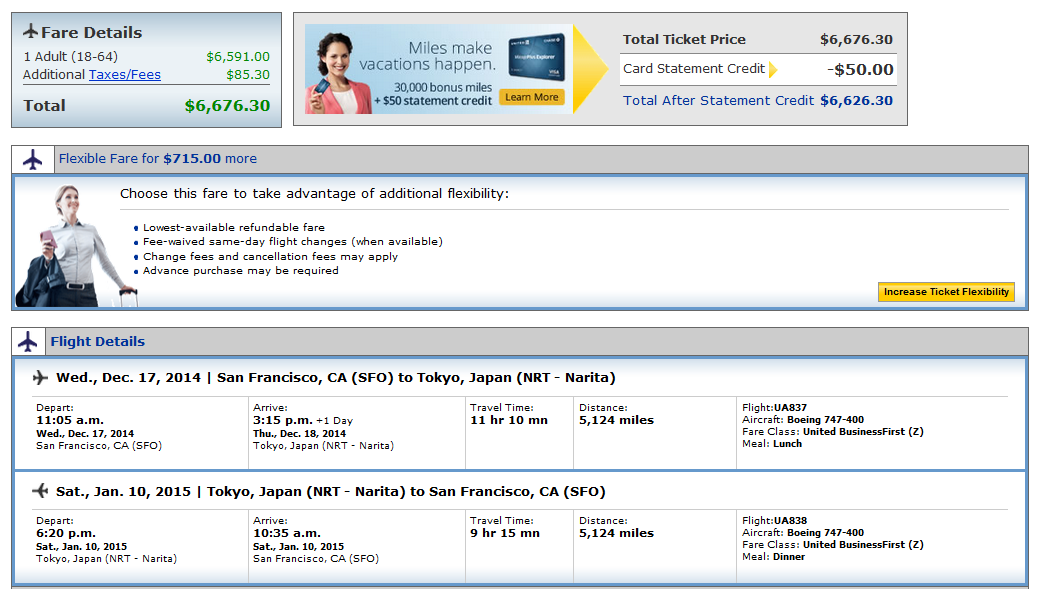**Screenshot of Web Page with Flight Details and Fare Options**

The screenshot captures a well-organized webpage with a clean white background, divided into three main sections.

**Top Section: Fare Details**
- **Background Color:** Baby blue
- **Graphic:** Black silhouette of an airplane in the top left corner
- **Text:**
  - **Title:** "Fare Details"
  - **Breakdown:**
    - "One Adult (18 to 64)": $6,591.00 (in green)
    - "Additional Fees (Taxes/Fees)": $85.30
  - **Total:**
    - In green, "$6,636.30" 

**Middle Section: Promotional Offer**
- **Background Color:** Baby blue
- **Graphic:** Image of a smiling woman of Caucasian European descent holding up a blue card. She wears a white shirt and a salmon-colored jacket.
- **Text:**
  - "Miles Make Vacations Happen"
  - Details of the credit card offer:
    - "30,000 bonus miles plus $50 statement credit"
    - Bold text in yellow arrow: "Total Ticket Price: $6,676.30"
    - "Card Statement Credit: -$50.00"
    - In blue: "Total After Statement Credit: $6,626.30"

**Bottom Section: Flexible Fare Option**
- **Background Color:** Baby blue
- **Graphic:** Image of a blonde woman of Caucasian European descent, holding rollaway luggage in her left hand while looking up and holding a phone and a blue jacket in her right arm.
- **Text:**
  - "Flexible Fare for $715 more"
  - Description:
    - "Choose this fare to take advantage of traditional flexibility."
    - Covers benefits such as the lowest available refundable fare.
  - **Button:** Large yellow button at the bottom right labeled "Increase Ticket Flexibility" in black.

**Footer Section: Flight Details**
- **Background Color:** Baby blue
- **Graphic:** Image of an airplane
- **Text:**
  - "Flight Details"
  - Departure and arrival times
  - Route: San Francisco to Tokyo